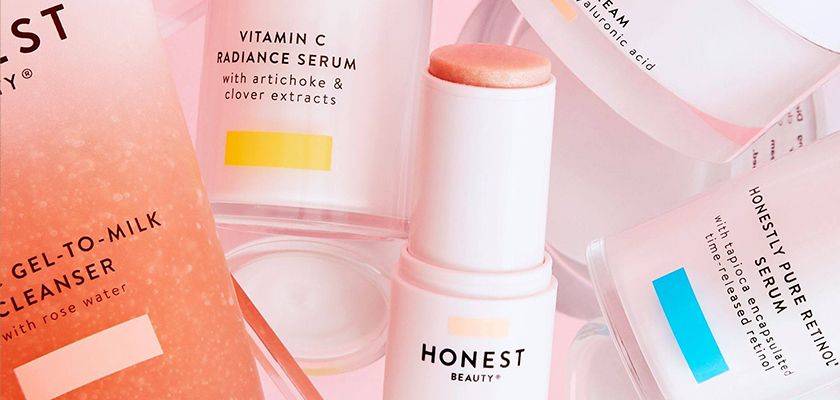The close-up image showcases a vibrant array of beauty products, crowded into the frame with no visible background. These products, primarily within the skincare and makeup category, are irregularly scattered and overlapping, giving it a promotional aesthetic. Central to the composition is an Honest Beauty tube with a creamy pink lid set aside, suggesting it might be a blush or similar product. Immediately to its right lies an Honest Beauty Pure Retinol Serum container, identifiable by a prominent blue stripe and text detailing its tapioca encapsulated time-release formula. Adjacent to this, a bottle filled with a pink liquid is labeled as a Gel-to-Milk Cleanser with rose water, distinguished by a white strip at its base. A Vitamin C Radiant Serum with artichoke and clover extracts is also prominently featured, with its text partially visible behind other products. The spectrum of colors in the image includes pink, orange, yellow, blue, white, and black, contributing to the dynamic and lively presentation typical of a beauty advertisement.